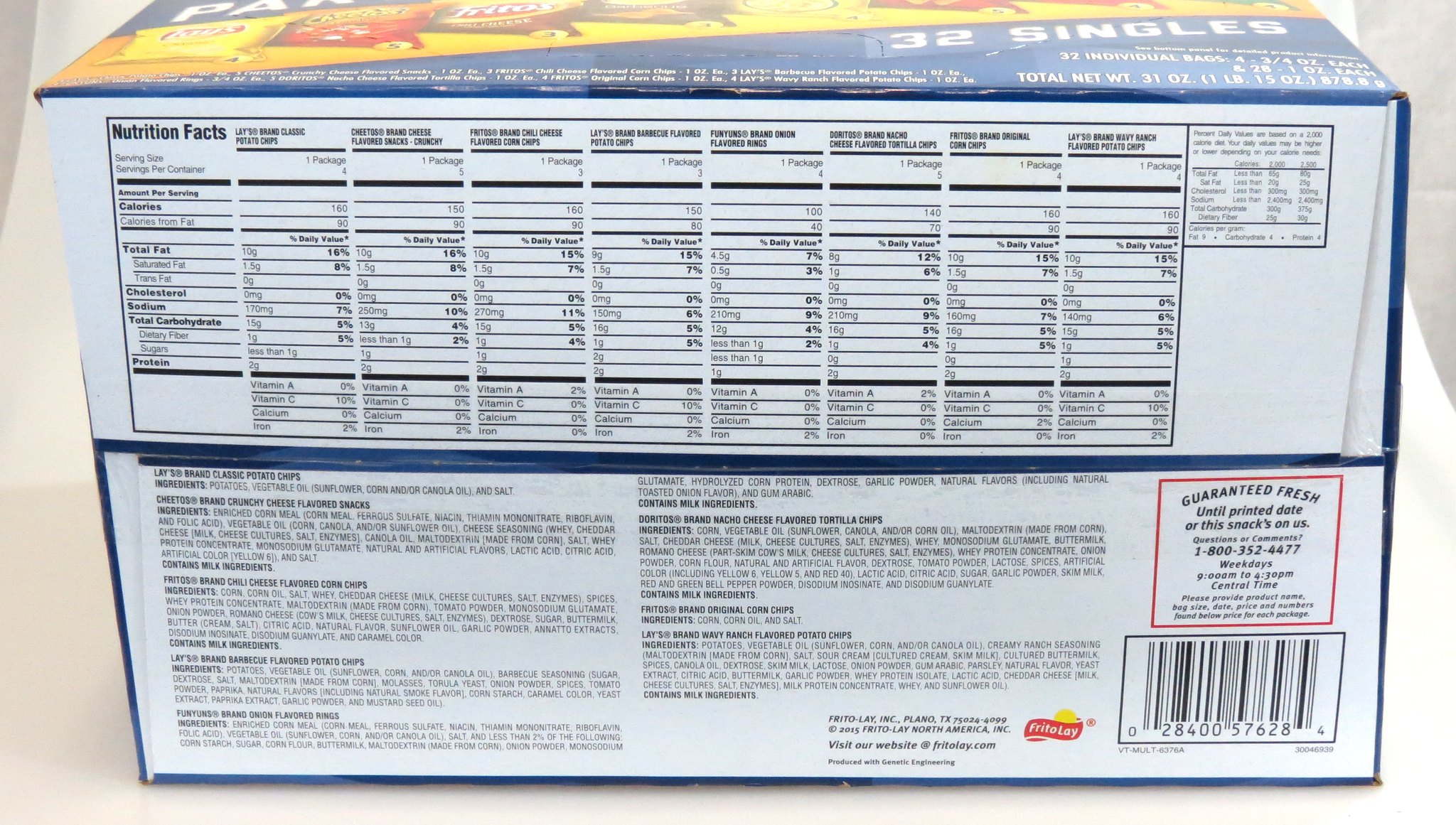The image displays a package of snacks on a white surface. At the top of the package, there is a blue section. The front prominently features the text "Nutrition Facts." Below the blue section, there is an assortment of snack chips with the label "32 Singles." Further down, black text appears, and there are multiple small squares and lines, indicating additional information and design details on the package. The right side has even more text. On the top right corner, there is a square section that includes a red button with the "Frito Lay" logo, and text that guarantees freshness until the printed date. Additionally, a phone number begins with "1-800-3..." but is not fully visible. At the bottom of the package, there is a barcode with the number "02840057628." The overall image is quite out of focus, making finer details difficult to discern.